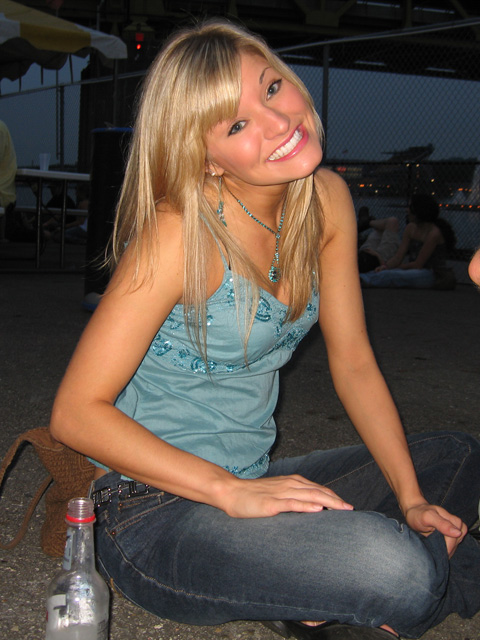In this nighttime scene, a young woman sits cross-legged on what appears to be a concrete surface, possibly near a roadway or a sidewalk, with a general ambience of a casual outdoor gathering. She is dressed in dark blue jeans and wears a teal tank top with thin shoulder straps, complemented by a matching blue necklace. Her long blonde hair cascades down to her mid-arm as she tilts her head slightly, smiling warmly at the camera, her pink lipstick accentuating her cheerful expression. The setting features a mix of elements: behind her is a chain link fence, and to the side, there's a white and yellow umbrella, suggesting the presence of a table nearby. Adding to the scene's casual vibe, a bottle rests on the ground in the lower left-hand corner, possibly an open soda. Her tan complexion and made-up face, featuring hazel eyes, are illuminated by the camera flash, highlighting the darkness around. In the background, red and white lights, along with elements like a brown purse and the dim outlines of what could be boats or water, hint at a lively, possibly beach-side gathering.